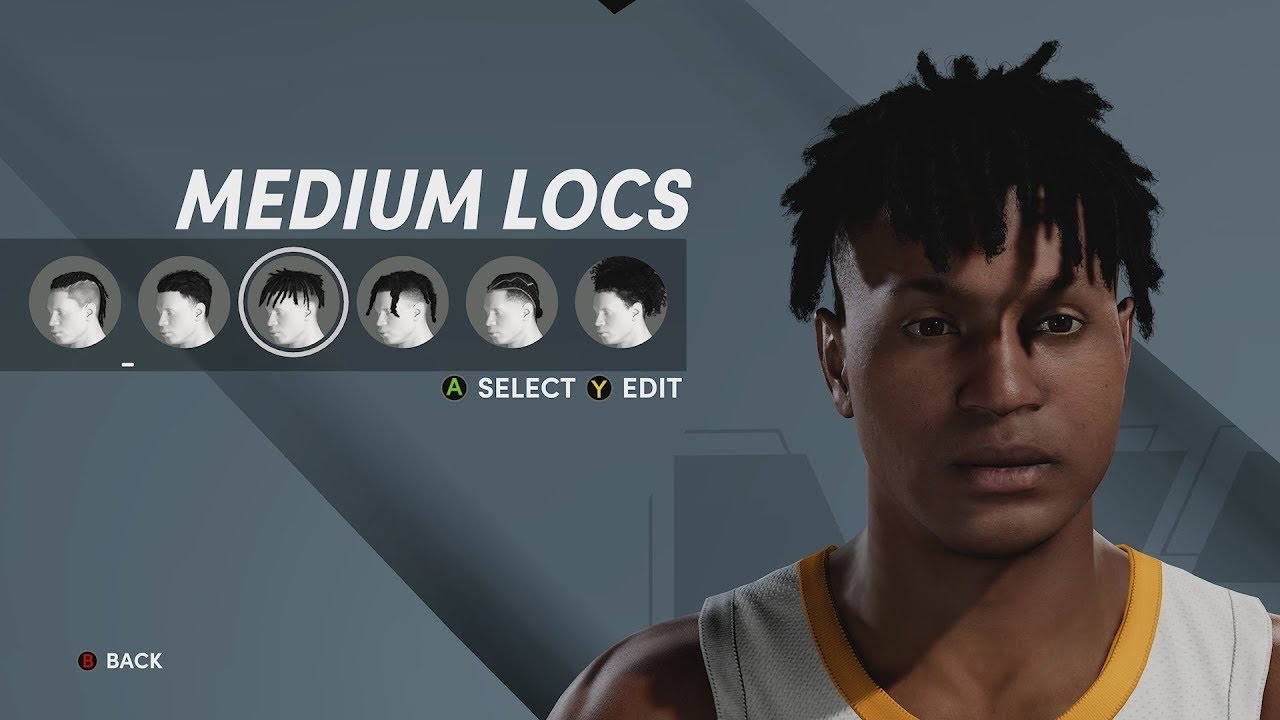In this detailed image, we observe the character creation screen of a sports video game, likely a basketball game. The primary focus is on the hair customization options for the avatar. The interface has a gray background, with the customizable player avatar displayed prominently on the right side of the screen. The avatar appears to be a Black male athlete, dressed in a sleeveless basketball jersey, indicative of the sport.

The character is currently sporting a hairstyle labeled as "Medium Locks," demonstrated by the dreadlock hairstyle on the avatar. On the left side of the screen, the hair customization menu is visible, displaying six different hairstyle options. The selected option, “Medium Locks,” is the third from the right in this lineup. Beneath the hairstyle options, there are control instructions: pressing 'A' to select a hairstyle and pressing 'Y' to edit further. This detailed arrangement allows users to personalize the appearance of their in-game character effectively.